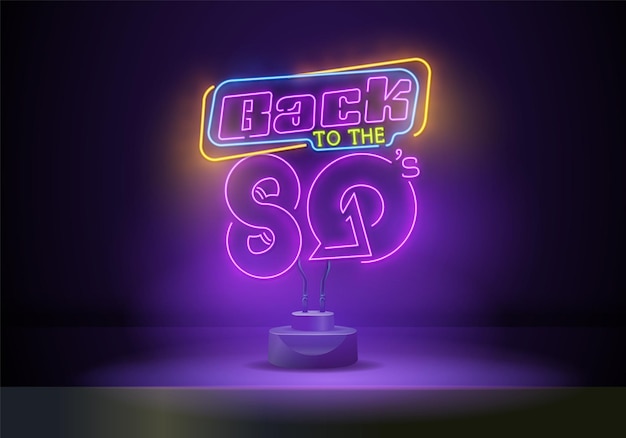The image depicts a vibrant neon sign illuminated against a black background atop a cylindrical, geometrically styled, two-level stand. The sign reads "Back to the 80s" in a playful, quirky font. The word "Back" is highlighted in a bright purple neon, "to the" is written in a striking neon green, and "80s" in the same eye-catching purple bubble font, with the "0" cleverly designed as a triangle/arrows pointing counterclockwise. Surrounding the text, a dual border frames the words: the inner border is a soft blue light, and the outer one is a radiant yellow, creating a captivating, multi-colored glow. The stand itself is composed of two concentric circular levels, providing a stable base for the sign. Thin electrical wires are discreetly visible, running up the left side, energizing the sign, and trailing back down on the right. The overall effect is a nostalgic, vividly luminescent tribute to the 1980s, highlighted by the rich purplish hue that pervades the setup.